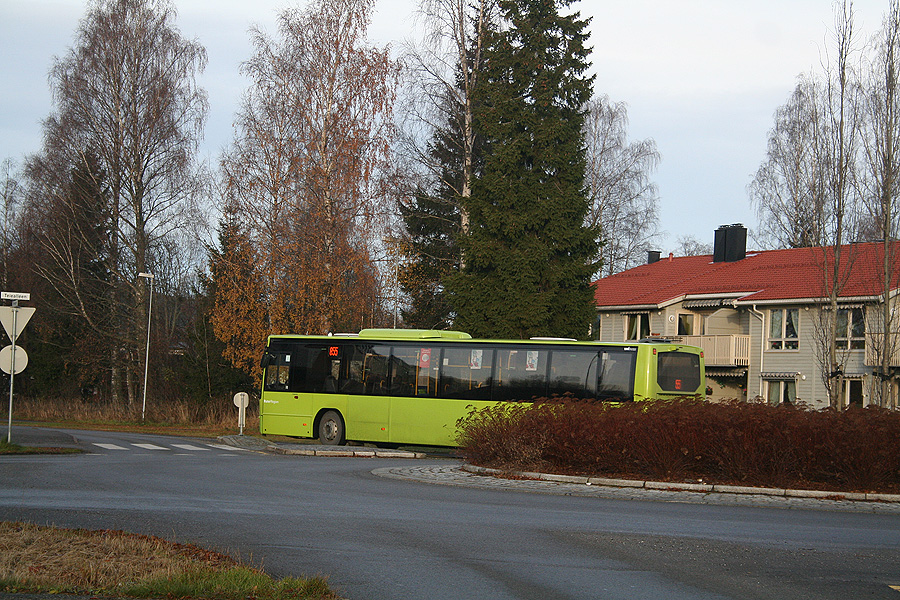This photograph captures a suburban or rural scene featuring a prominent roundabout intersection. At the focal point of the roundabout, there is a landscaped center island with a large hedge and some dried plants, indicative of an autumn setting. Surrounding the roundabout are various trees, including a tall evergreen and few others with reddish leaves or almost bare branches.

Dominating the mid-ground of the image is a large, lime green city bus with expansive black windows, traveling from the right to the left side of the frame, seemingly making its way through the roundabout. 

In the background, to the right of the bus, stands a double-story townhome or small hotel. This building has a red, angled roof, tan siding, numerous windows, and possibly individual balconies or diverse rooms indicated by various curtains. Additional street elements include visible street signs and possibly a streetlight, enhancing the urban feel of this intersection scene.